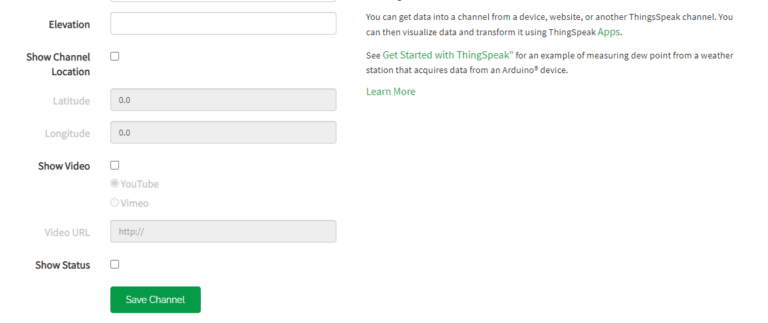The image depicts a partially scrolled website, likely belonging to ThingSpeak, a service platform for IoT analytics. On the left side, there is a menu where users can input elevation details. Additionally, there are options to display the channel location by specifying latitude and longitude coordinates. The interface includes a clickable 'Show Video' button, and it appears the user has selected YouTube for video integration, as opposed to Venmo. A URL input field is visible with a sample HTTPS address, likely representing a video link. Other elements in the menu include a 'Show Status' option and a prominent green 'Save Channel' button.

To the right, the interface offers guidance on data integration, suggesting that data can be imported into the channel from a device, website, or another ThingSpeak channel. It explains that users can visualize and transform the acquired data using ThingSpeak applications. An example use case for the platform is provided, highlighting how to measure dew point using a weather station that collects data from an Arduino device. The text also encourages users to learn more by exploring how to get started with ThingSpeak.

Unfortunately, the top section of the website is not visible in the image, leaving the exact nature of the page somewhat unclear. However, the description and examples provided strongly imply that the website is indeed ThingSpeak.